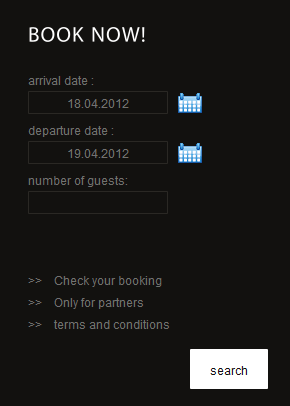The image is a screenshot from a travel website displayed on a mobile device in portrait mode, set against a black background. At the top left corner, in all capital white letters, is the text "BOOK NOW!" Directly beneath this prompt, in lowercase text, it indicates "arrival date:" followed by a white outlined rectangle displaying the date "18.04.2012" (April 18th, 2012). To the right of this date field is a clickable blue and white calendar icon designed to allow users to select their arrival date. Below this is another similar white outlined rectangle labeled "departure date:", showing "19.04.2012" (April 19th, 2012), again with a blue and white clickable calendar icon to the right.

Further down is the text "number of guests" with an empty outlined rectangle below it, which is black inside, indicating that no number of guests has been entered. This field does not appear to have a drop-down menu, requiring users to manually input the number of guests.

Toward the bottom of the screen are three rows of text, each prefaced with double right-pointing, nested open arrows. The first row says "Check your booking," with "Check" starting with a capital C. The second line reads "Only for partners," capitalizing the O in "Only." The third and final row states "terms and conditions" entirely in lowercase letters.

In the bottom right corner, there is a white clickable button labeled "search."